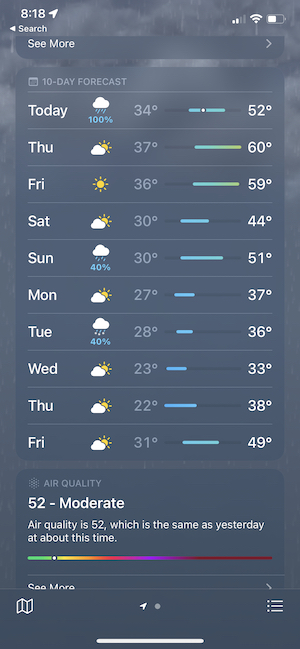This image shows a device screen with detailed information and various icons. In the top-left corner, the time is displayed as 8:18, next to a GPS icon on the right. On the top-right, there are three icons: a cellular signal icon, a Wi-Fi signal icon, and a battery icon. Immediately below the time, the word "Search" is visible, followed by the phrase "See More." The main content of the screen features a title reading "10-Day Forecast," under which the days are segmented by white lines.

The first section is labeled "Today" and displays a cloud icon with rain, indicating a 100% chance of precipitation. Next to this, the temperature range is shown, with a low of 34 degrees and a high of 52 degrees. Below this, the forecast for "THURS" (Thursday) includes a cloud and sun icon with a temperature of 37 degrees. Further down, the forecast for "Friday" is indicated.